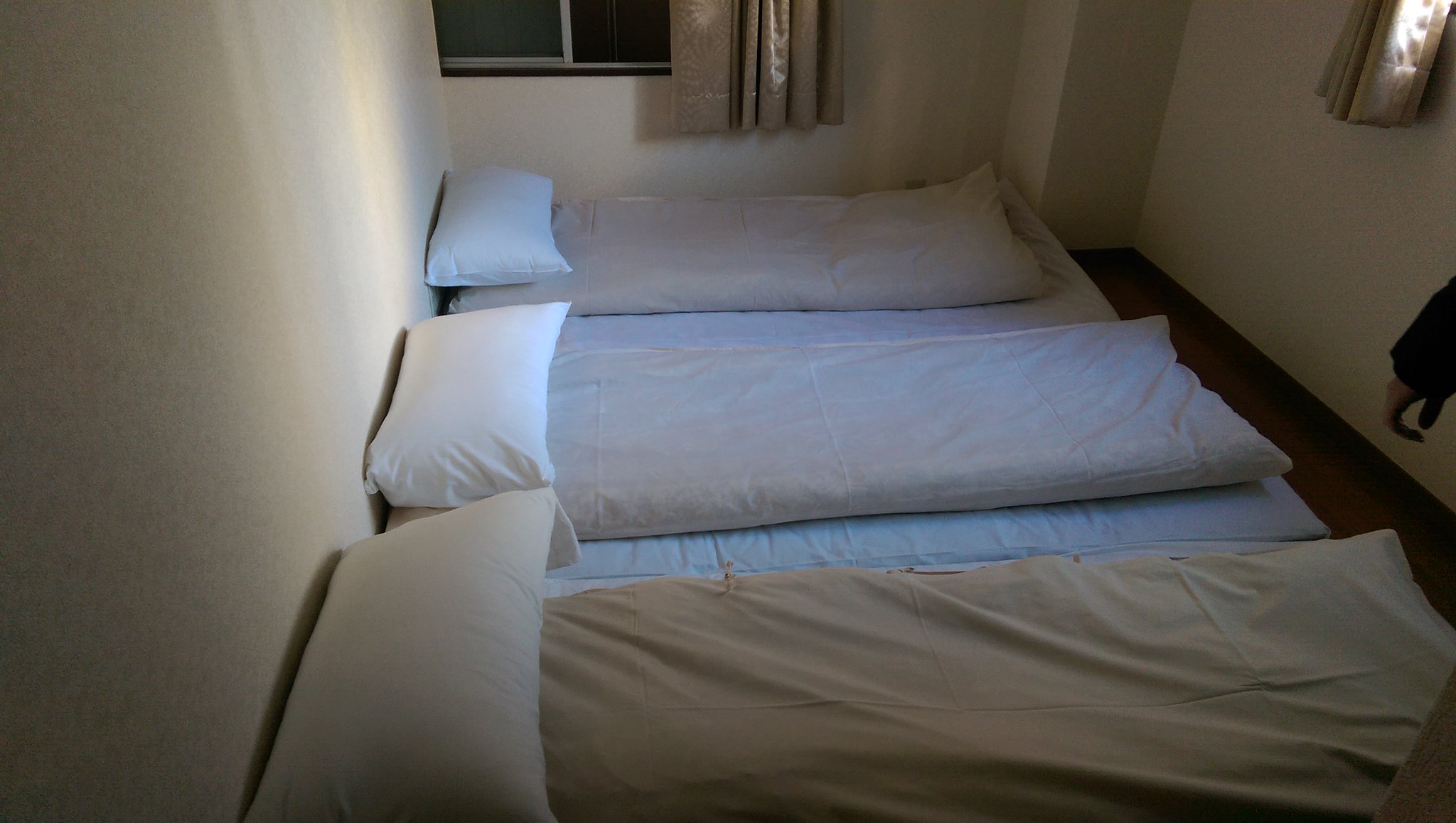The photograph captures the inside of a narrow, long room with stark, tan-colored walls and a dark floor. Three makeshift beds, low to the ground, stretch across the entire length of the room. Each bed consists of a comforter folded in half acting as a mattress, a white pillow at the top, and a blue blanket underneath. Additionally, every bed is topped with a sleeping bag. The room features two windows, each with beige curtains that are partially open, allowing light to filter in. On the right side of the image, a man's left hand and wrist are visible, dressed in a black coat, adding an element of mystery to the otherwise sparse and utilitarian setting.